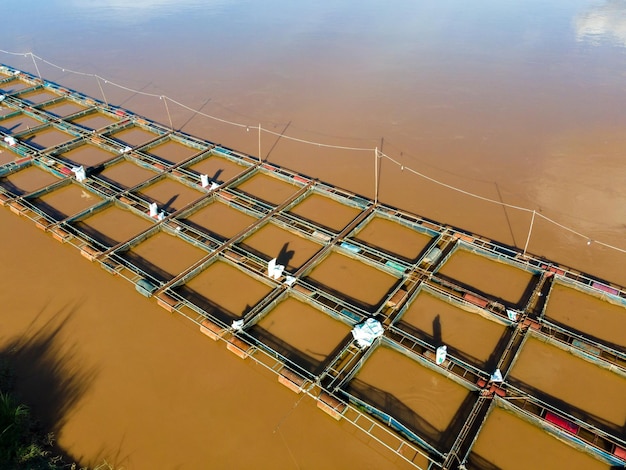The image depicts a stark and dreary scene of a large, floating grid structure set in a vast expanse of murky, muddy brown water, possibly a slow-moving river or a large lake. The grid, seemingly made of gray metal, is divided into numerous rectangular compartments and is buoyed by an array of 50-gallon drums of varying colors—predominantly tan, light blue, with some brown and red. The structure stretches diagonally from the bottom right to the upper left of the photograph. Reflections of the sky with a few clouds are visible along the top edge of the picture, while a shadow is noticeable in the bottom left corner. To the far right, a line—potentially electrified—supported by poles runs parallel to the structure, which might be used for lighting. The overall appearance suggests it is part of a fish cultivation operation for the food market, emphasizing the pragmatic and industrial aesthetic of the scene.